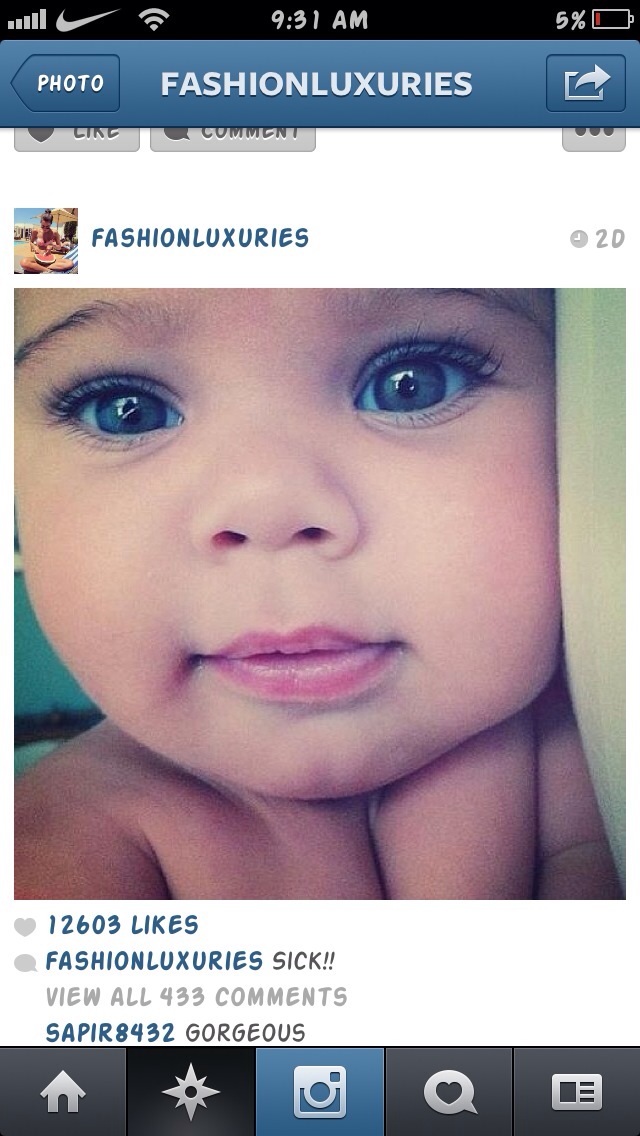The image is a screenshot of a social media page, likely from an older version of Instagram. At the top of the phone screen, icons indicate it's 9:31 AM, with 5% battery remaining, full Wi-Fi signal, and phone connectivity. The page loaded belongs to "Fashion Luxuries," identifiable by a blue bar header featuring the account’s name. The profile picture for Fashion Luxuries is a square icon showing a woman in a bikini eating something, possibly scooping a watermelon. Below this, the main content is a close-up photo of a baby girl with striking features: large, bright blue eyes, long eyelashes, and pink lips. Her skin has a light tan hue, and her eyebrows are dark. The post by Fashion Luxuries has garnered 12,603 likes, and the caption reads "sick!!!" One visible comment by a user named Sapiri8432 simply says "gorgeous." At the bottom, the Instagram footer indicates options like the home screen and post screen.